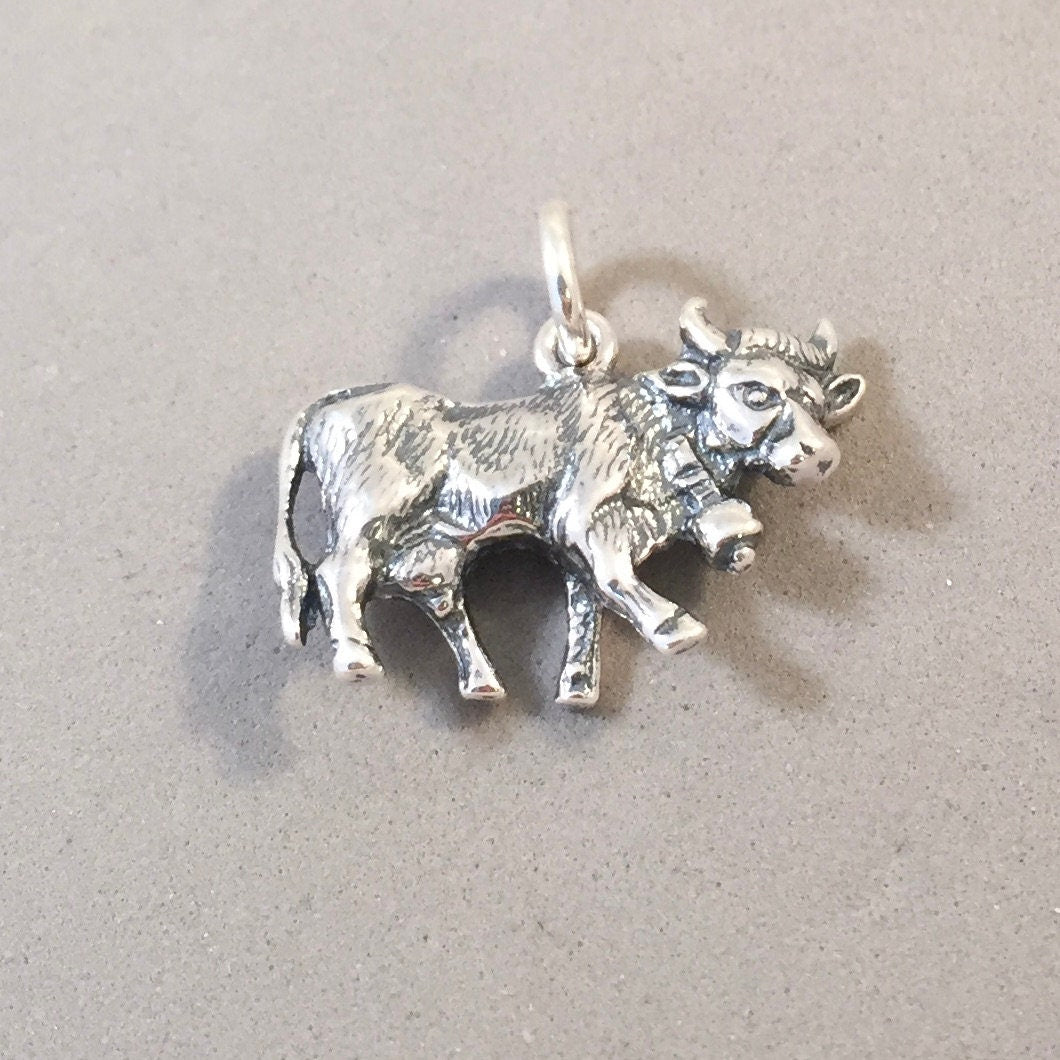This image showcases a square-shaped photograph of a small, silver-colored pendant designed as a cow. The pendant is crafted either from pewter or silver, highlighting meticulous details such as the cow's feet, fur, and a cowbell around its neck. Notably, the cow's head features distinct horns, eyes, ears, nose, and mouth, with one of the ears appearing twisted and almost wrapping around its eye. The cow’s stance shows one hoof lifted, while the other three remain grounded. The pendant includes a loop for attachment to a necklace or bracelet, emanating a slight shadow on the textured, granite-like surface beneath it. The background is a beige-ish light gray with faint speckles in black and white, contributing to the image’s detailed composition. The pendant’s shadow suggests the light source is positioned above, further accentuating its proportional yet slightly exaggerated features, such as the elongated tail nearly spanning the cow’s entire height.